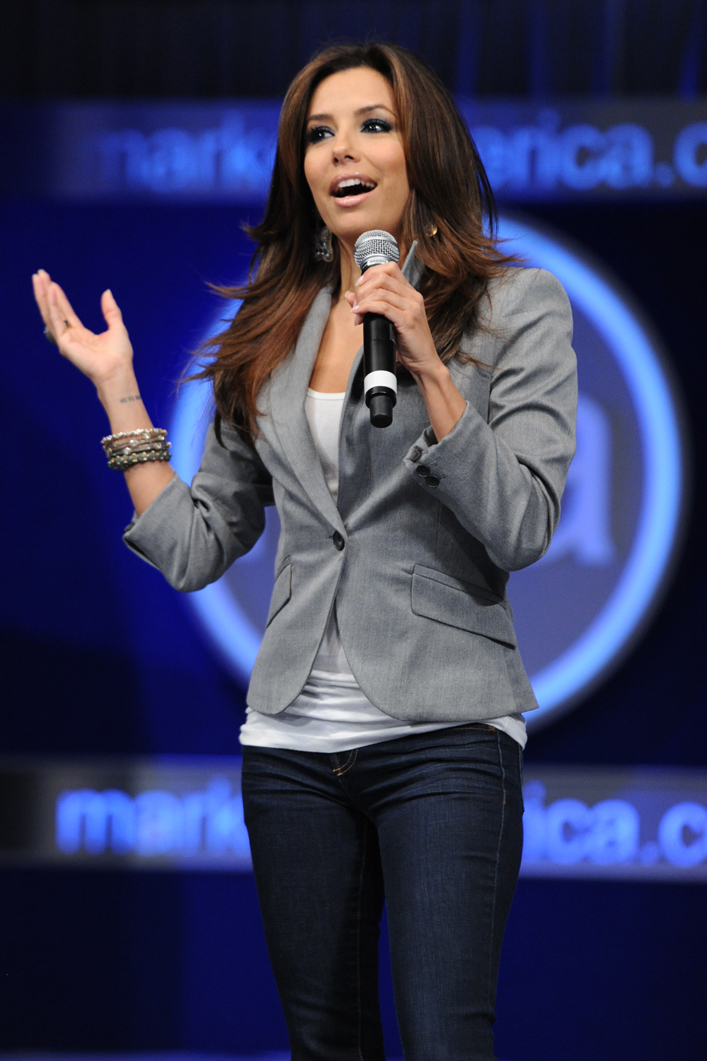In this indoor image, a woman resembling Eva Longoria stands confidently at the center, holding a silver and black microphone in her left hand while mid-sentence. She is dressed in blue jeans, a gray sports jacket over a white blouse, and has a round necklace on her lower right hand. Her brown, slightly reddish hair cascades down as she extends her right arm, hand bent upwards. The blurred background features some indiscernible text or poster in shades of dark, light blue, and black. The colors in the scene notably include black, blue, white, gray, tan, and silver. The photograph hints at a speaking event or presentation.